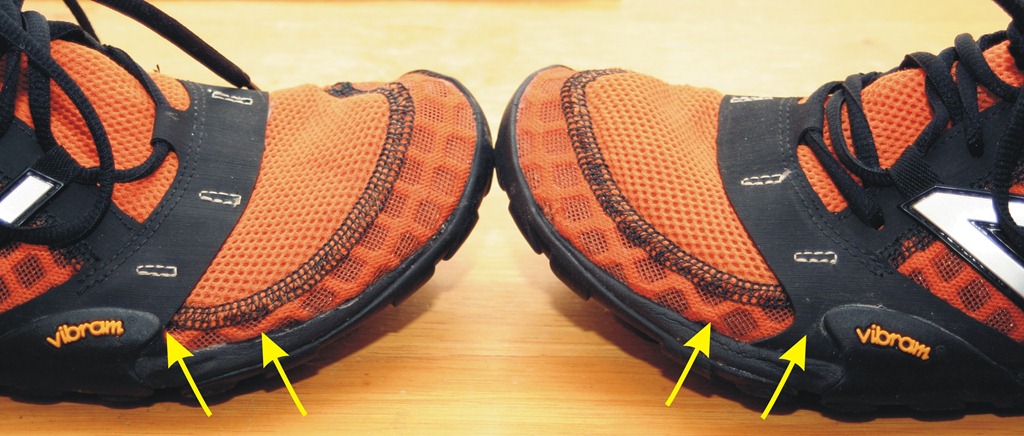This image features a wide, horizontally-aligned rectangular photograph of a pair of orange shoes, positioned toe-to-toe in opposite directions on a light brown wooden floor. The right shoe extends from the left side of the image, showing its front half, while the left shoe extends from the right, similarly revealing only its front half. Both shoes are crafted from an orange fabric, likely canvas, and adorned with black shoelaces and a prominent black fabric segment crossing over the upper portion, just past the toes but stopping short of the shoelace area. The soles are made of black rubber. The brand name "Vibram" is printed in orange on the black segment on both shoes. Additionally, a white upside-down V-like logo is partially visible on the right shoe. Two small yellow arrows on each shoe point towards distinct sections, presumably indicating the black segment where the brand name is written and the orange fabric part.